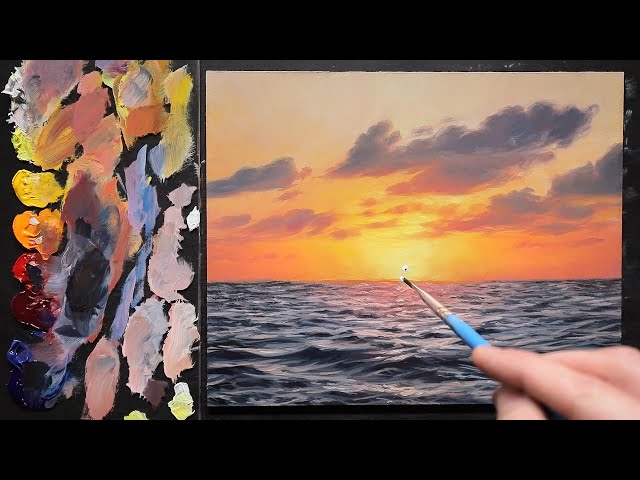In this image, an artist is engaged in painting an ocean landscape against a plain black background. To the left, there is an easel with a palette displaying a variety of colors, including white, yellow, orange, red, purple, and blue, meticulously mixed in gradients. The painting being created, prominently situated on the right, depicts a serene sunset or sunrise over a vast body of water. The sky is illuminated with vibrant hues of yellow and orange, blending beautifully into the clouds drifting across it. Below, the ocean is depicted with a darkish blue hue, filled with intricate ripples. The artist's hand, although slightly out of focus, is visible holding a fine paintbrush with a blue handle, tipped with white paint, poised to add delicate details to the radiant sun at the center of the canvas.